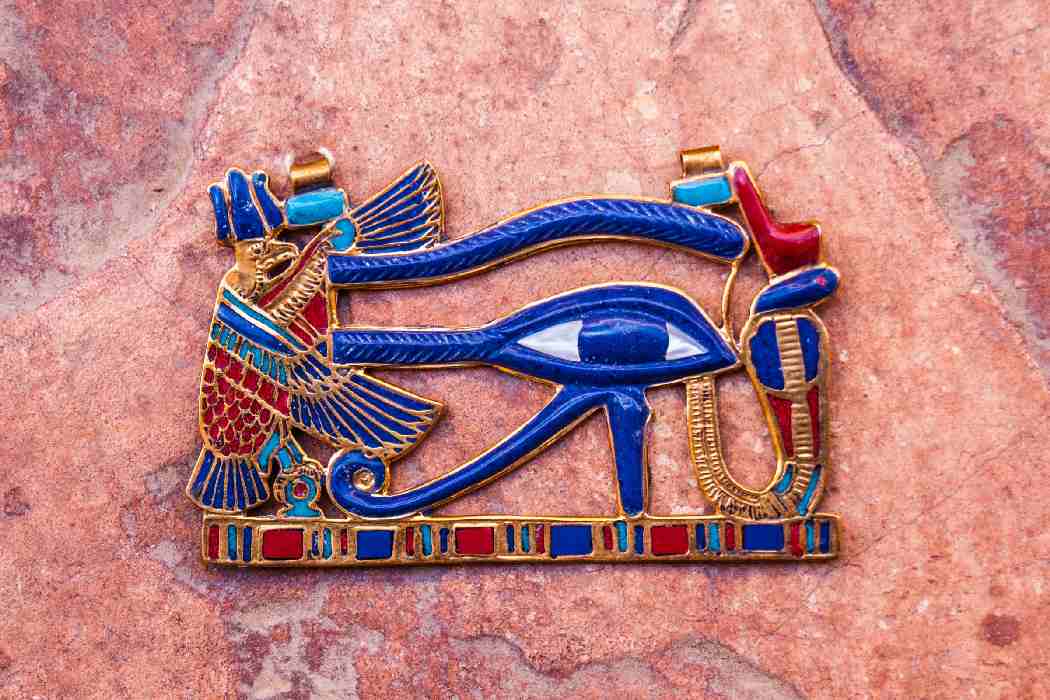The image depicts a meticulously detailed and well-preserved representation of an ancient Egyptian-inspired emblem. Set against a horizontally oriented background of red bricks or red stone, the central focus is a striking blue eye symbol, adorned with intricate golden trim and multicolored decorations. This eye, possibly representing the Eye of Horus, is flanked on the left by a vibrantly colored eagle with blue, red, and gold feathers. The eye itself is detailed with two horizontal lines crossing it and an intricate upside-down check mark with decorative swirls beneath. To the right of the eye are additional decorative swirls, contributing to the emblem's ornate design. Surrounding the eye and bird are patterns of small cylindrical shapes alternating in red and light blue, interspersed with larger squares and rectangles, creating a visually captivating border. The emblem appears either exceptionally well-preserved or a high-quality reproduction, possibly intended as a brooch or a necklace pendant, identifiable by the loopholes at the top for hanging. This elaborate creation showcases a blend of ancient artistry and symbolism, evoking the timeless aesthetic of Egyptian culture.